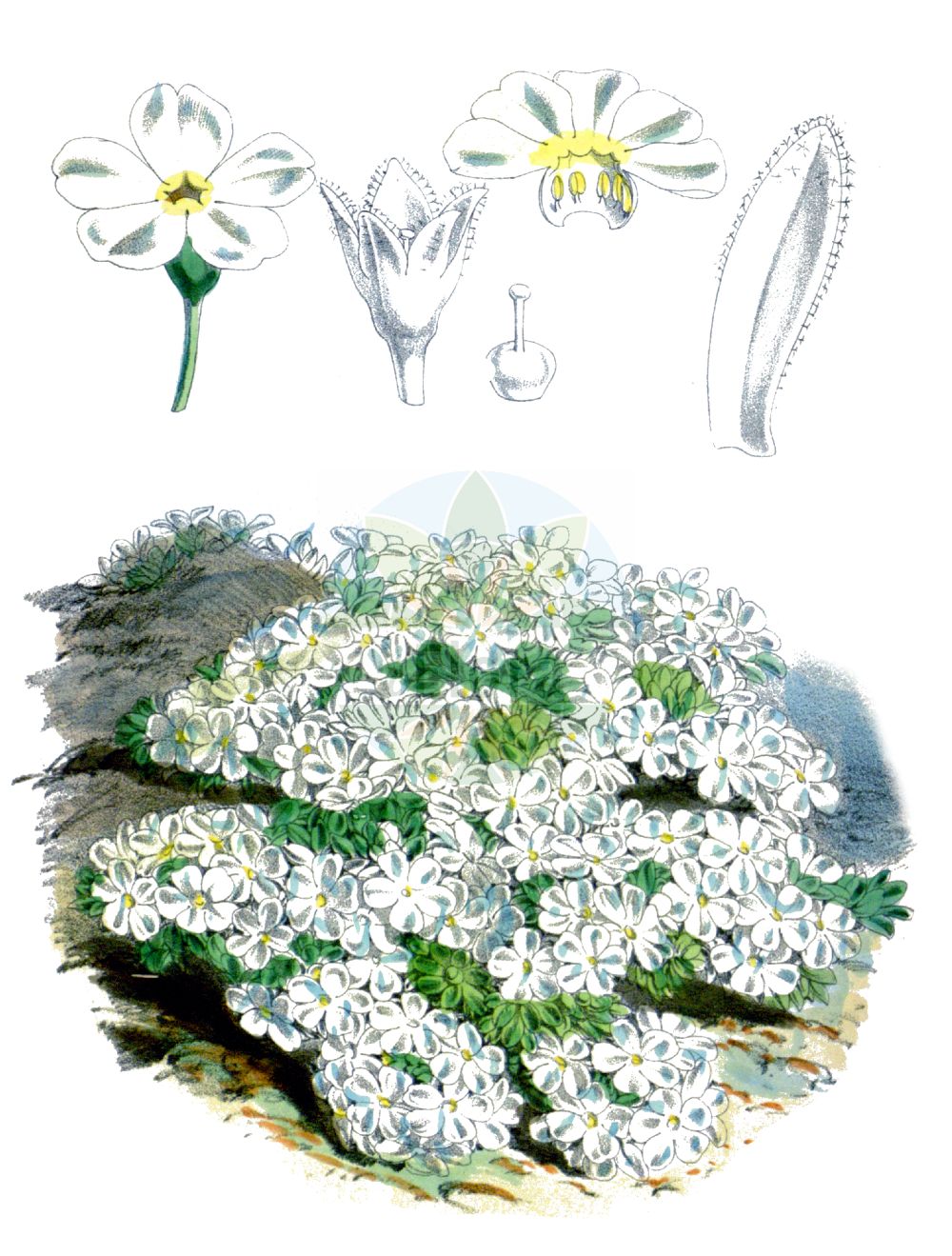The image is a detailed botanical drawing featuring a circular artificial bouquet of small white flowers with green leaves at the bottom. The bouquet is intricately composed with a realistic depiction, showing a dense cluster of flowers arranged in a bush-like formation. Above the bouquet, the drawing meticulously breaks down and showcases individual parts of the flower starting from left to right. You see a fully bloomed white flower with five petals and a yellow center attached to a green stem. Next is an illustration of the flower in its bud stage with upright small petals. This is followed by a round bulb with an antenna-like structure topped with a ball. Further to the right, there's a depiction of the top half of the yellow core with yellow seeds, and next to it, a single elongated, curvilinear petal with lines possibly indicating pollination. All individual flower components appear on a white page, presented in a systematic manner to detail the construction of the flower meticulously.